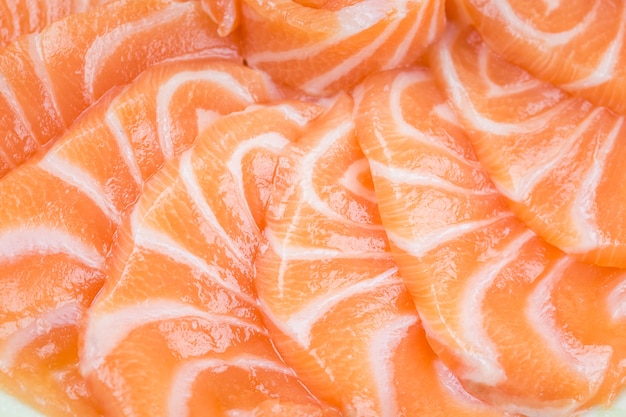The image features thinly sliced pieces of salmon, arranged in a visually appealing pattern. The salmon flesh exhibits a distinctive orangey-pink hue with intricate white marbling, indicative of a fatty and fresh cut. The delicate slices are arranged in a swirling, decorative fashion, almost resembling the intricate icing on a cake or the layered presentation of thinly sliced fruits like peaches or oranges. This sashimi-style presentation showcases the moist, succulent texture of the salmon, which could be enjoyed raw with a light squeeze of lime and other seasonings, emphasizing its sushi-quality freshness.